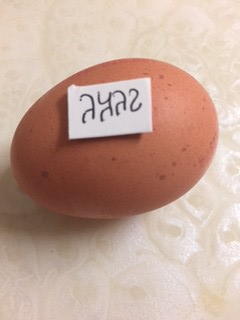The photograph captures a brown chicken egg with a teardrop shape, positioned on its side on a textured white surface that has a pearly shine. The narrower top of the egg points to the left, while the wider bottom points to the right. The egg, which some describe as having a color almost like a potato, is adorned with various dark brown speckles. Adding an intriguing element, a small rectangular piece of white paper is affixed to the middle of the egg. This paper bears four handwritten characters in black ink that resemble symbols rather than recognizable letters or languages. The overall image composition places the egg at the center, highlighting its unique details against the backdrop that could be a tablecloth or another textured material.